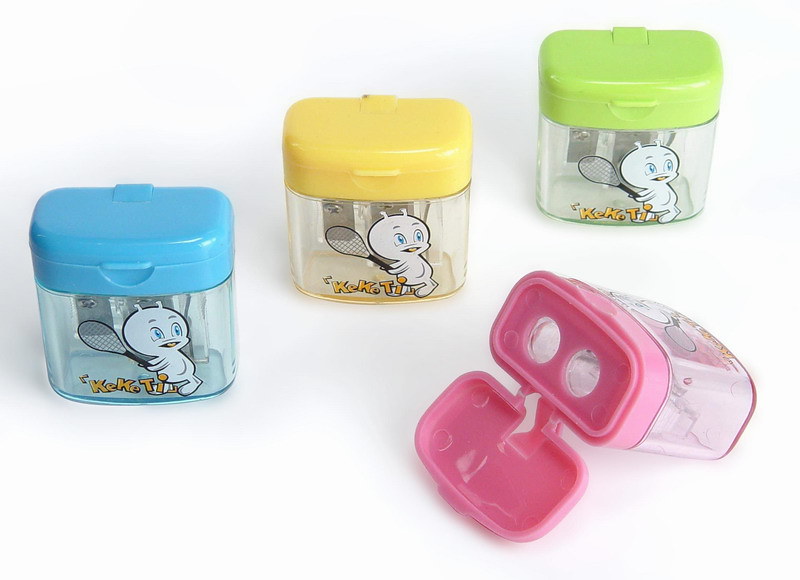In the photograph, there are several plastic pencil sharpeners, each featuring the same whimsical image of a white alien cartoon character with blue eyes, antenna, stubby arms, and legs, holding a tennis racket. The text "Kiki T" is printed in yellow on each sharpener. The sharpeners are identical in design but come in four distinct colors: pink, blue, yellow, and green.

Additionally, there are small bins designed to hold items, possibly snacks for infants, evident from their practical, clear bases and hinged, colored acrylic tops. The tops have flip-open lids, revealing two smaller circles inside, suitable for shaking out contents like Cheerios. The bins stand upright in blue, yellow, and lime green colors, while a pink one is positioned in the bottom right corner with its lid open, adding a practical demonstration of its functionality.